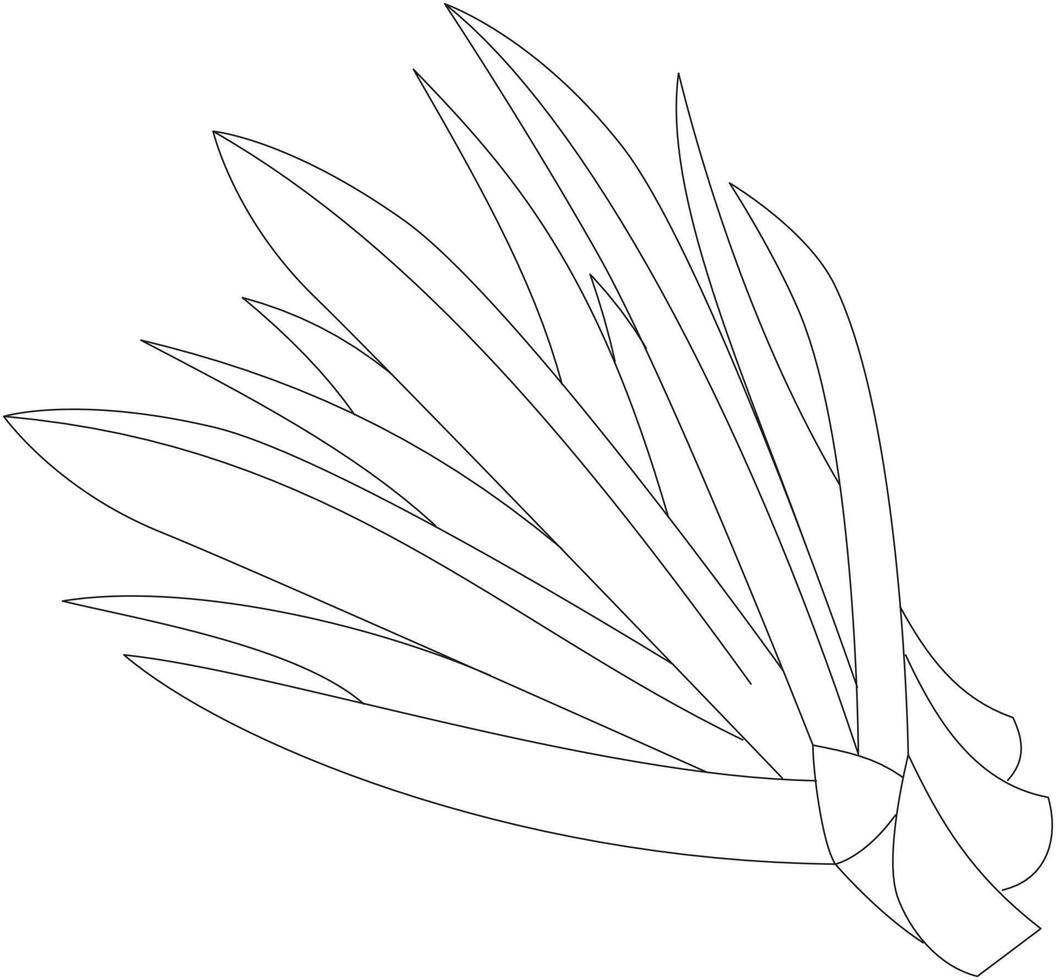This image features a black and white digital drawing resembling an abstract or stylized plant. Against a pristine white background, the plant-like figure emerges from a base in the lower right-hand corner, which appears to function as a handle. This base extends upward into a series of elongated, pointy leaves that diverge in multiple directions. Starting from the base, the leaves on the left side extend horizontally at a slight angle, while those on the right side project vertically. Central to the image, larger, blade-like leaves ascend and spread outwards, reaching towards the upper left, center, and upper right portions of the composition. The leaves are intricately detailed, emphasizing their elongated and sharp appearance, similar to a fern or plantain leaves drawn with fine ink lines or a digital pen. The absence of text allows the viewer to focus solely on the plant's elaborate structure and artistic form.